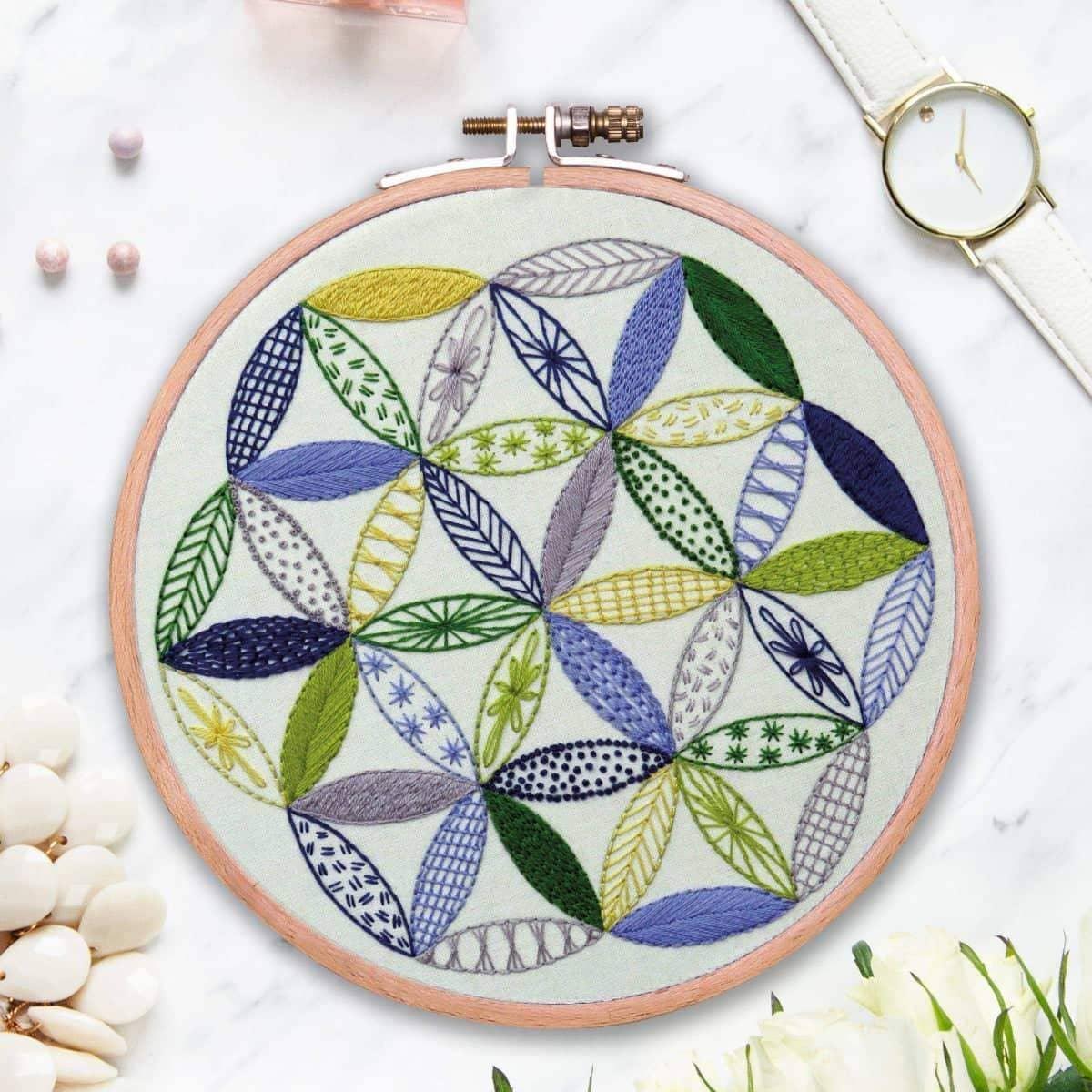This detailed photograph showcases a pink embroidery hoop positioned on a marble countertop. The clasp tightening the hoop is at the top, with its brass end facing to the right. The hoop frames a complex piece of embroidered artwork featuring an intricate geometric design of interconnected circles and triangular cells. The triangles are crafted from pointed ovals and filled with an assortment of patterns, including leaf-like veins, spokes, lines, and dots, in shades of dark blue, light blue, green, dark green, light green, yellow, light purple, and periwinkle.

Surrounding the embroidery hoop, additional items add texture and context to the scene. In the upper left corner, three pink beads are scattered, while the top left edge hints at the presence of a pink crystal. A gold-rimmed women's wristwatch with a white leather-like band is placed in the top right corner. White roses with green leaves radiate from the bottom right corner, offering a touch of natural beauty. On the bottom left, white stones accented with brown interspersed gaps can be seen, potentially representing a piece of jewelry. The white background within the hoop is part of the fabric used for the embroidery, with small segments extending outside the hoop, blending slightly with the marble backdrop.